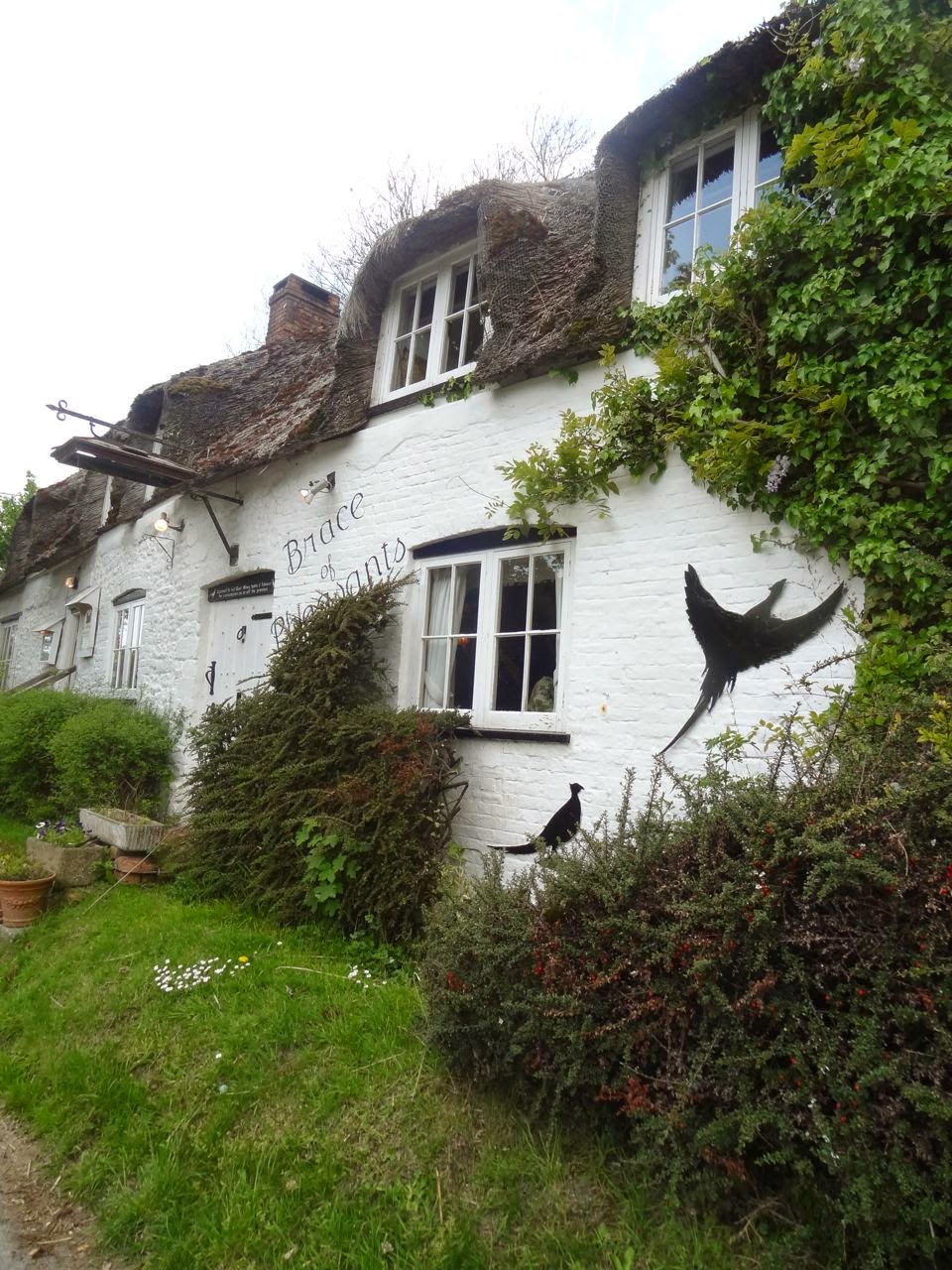The image depicts an old house situated in the countryside, possibly in England. The house is a white brick building with a thatched roof that gives it a rustic, European charm. A red brick chimney is visible atop the second story, which features gables. The frontage of the house is slightly sloped and covered in scraggly grass and scattered bushes, with some white flowers dotting the lawn and several planters with flowers leading up to the front door.

The building appears somewhat neglected, with ivy or other climbing plants growing up the side, displaying a gradient from darker green at the base to brighter green as it ascends. On the facade of the building, near the pathway, cursive writing spells out "Brace of Pheasants." Below this inscription, two metal silhouette artworks of pheasants are mounted on the wall—one bird is in flight, while the other stands still.

The structure's exterior is a blend of old charm and slight disrepair, hinting at a history that could involve hunting, hosting, or simply being an enduring countryside residence. The overall scene is enveloped in a tranquil, yet slightly unkempt rural atmosphere, portraying a picturesque, albeit weathered, slice of countryside life.